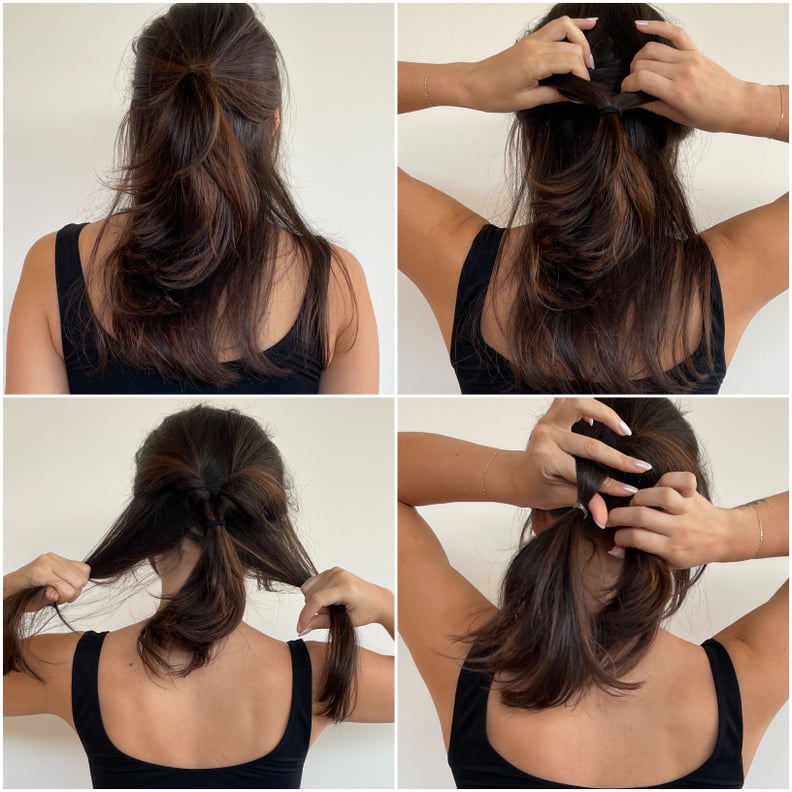The image is a detailed series of four photographs that guide viewers through the steps of creating a unique braided hairstyle. The model, a Caucasian woman with light skin and shoulder-length brown hair, is seen from the back in all stages. In the top left image, she begins with her hair pulled into a back ponytail while wearing a black tank top. In the top right image, she has her hands in her hair, separating it into sections. The bottom left image shows her pulling two strands of hair outward from each side, and finally, the bottom right image captures her twisting these strands around each other, creating a layered and textured braided look reminiscent of a princess style. The model's confident handling of her hair, despite not seeing what she's doing directly, highlights her skill and ease with the hairstyle.